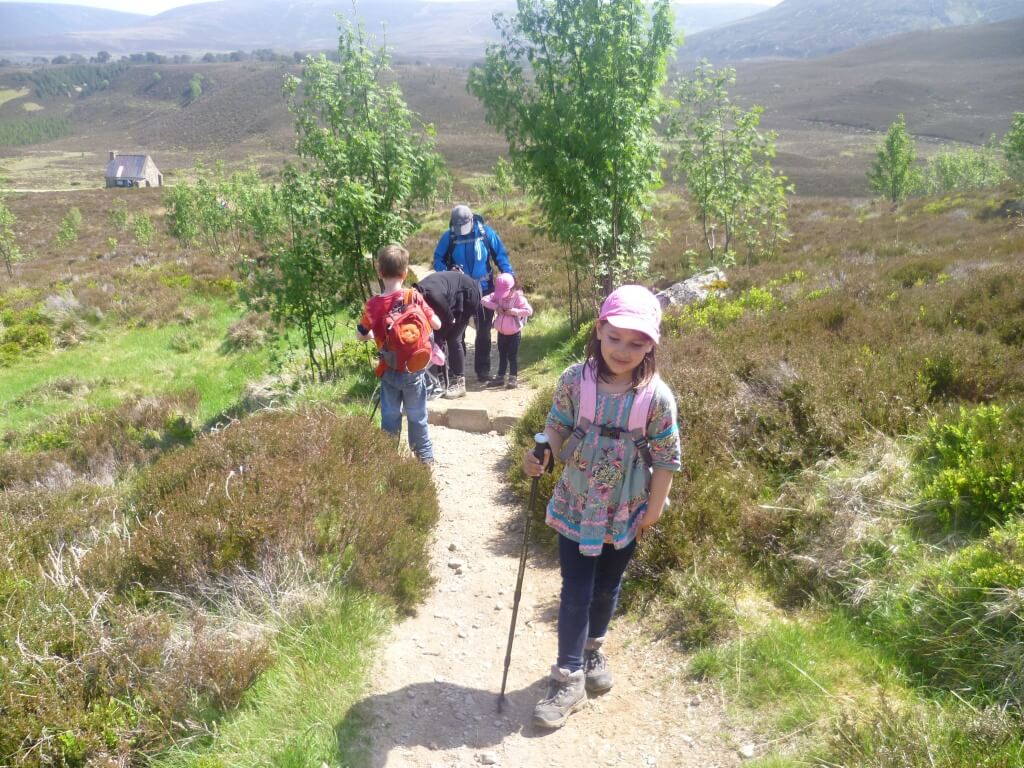The image depicts a semi-rural, farmland setting with a family, or possibly a school group, hiking along a nature trail. In the foreground, a young girl, likely around 10 years old, stands centrally, facing forward. She is dressed in a gray dress shirt, dark blue leggings, hiking boots, and a pink hat. She also carries a walking stick, which might be a support for sight or just part of her hiking gear. Flanking her on both sides are short trees and shrubbery, with visible rocks crossing the trail.

In the middle ground, the rest of the group comprises two adults and two more children—a boy and another girl. The boy wears a red shirt and a red backpack, and the girl, also in a pink hat, appears to be wearing similar hiking attire. The adults, who might be parents or teachers, are dressed in outdoor clothing, including a blue jacket and possibly a black hoodie. The trail they walk on is well-defined, with grassy and bushy terrain on either side.

The background reveals a hilly landscape, with mountains farther in the distance and a small house or shack perched in the upper-left corner, adding to the rural charm of the scene. The sun is shining brightly, suggesting it is either midday or later in the afternoon. The vibrant colors present in the image include pink, blue, red, orange, green, brown, gray, black, and white, enriching the picturesque rural environment.